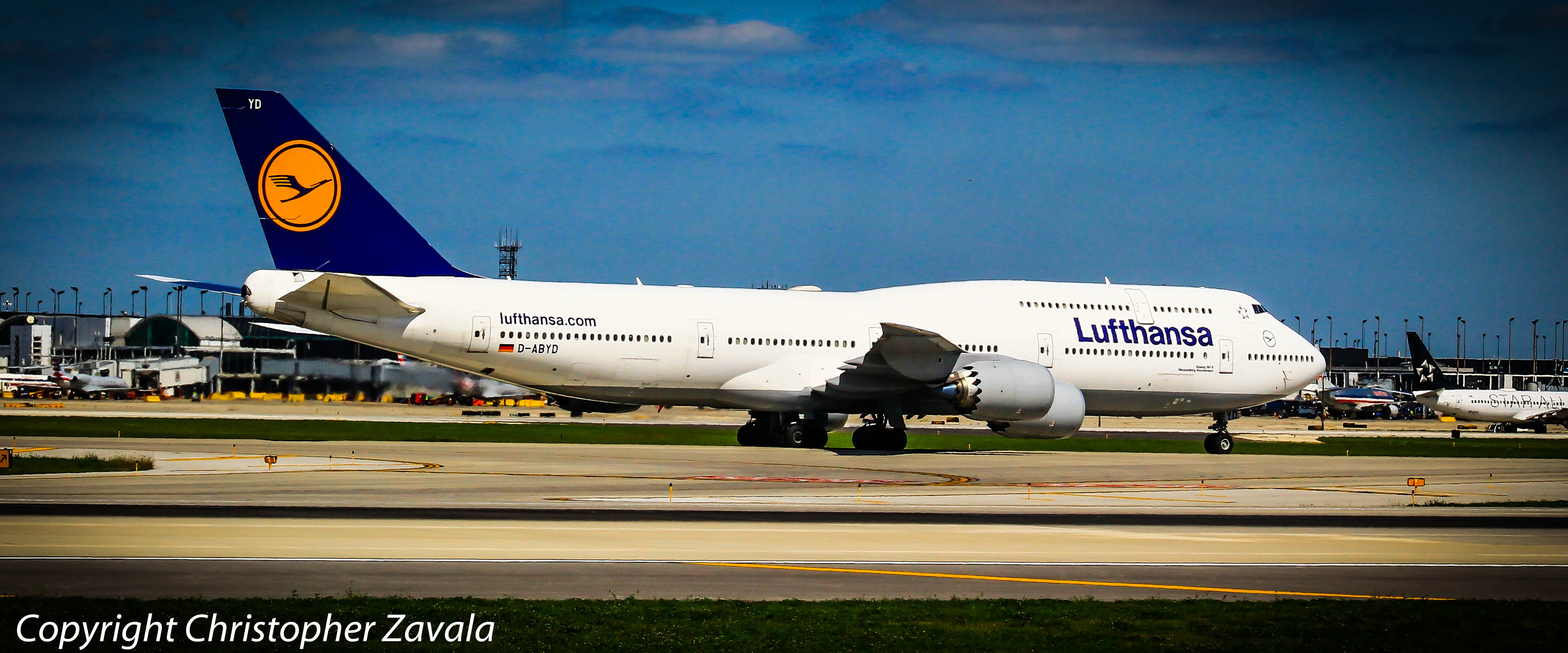The photograph, taken by Christopher Zavala, captures a Lufthansa Boeing 747 aircraft on a sunny day with a few clouds scattered in the blue sky. The image is horizontally oriented, showcasing the aircraft in a side view on a gray runway with yellow stripes. The white jetliner, bearing the blue and gold Lufthansa emblem on its tail, which also displays the registration "D-ABYD", takes center stage. The name "Lufthansa" is prominently visible near the front of the plane. The background reveals airport buildings, several vehicles, tall streetlights, and other planes waiting on the tarmac. The bottom corners of the photo feature a subtle gray gradient, with "copyright Christopher Zavala" elegantly italicized and positioned at the bottom left.